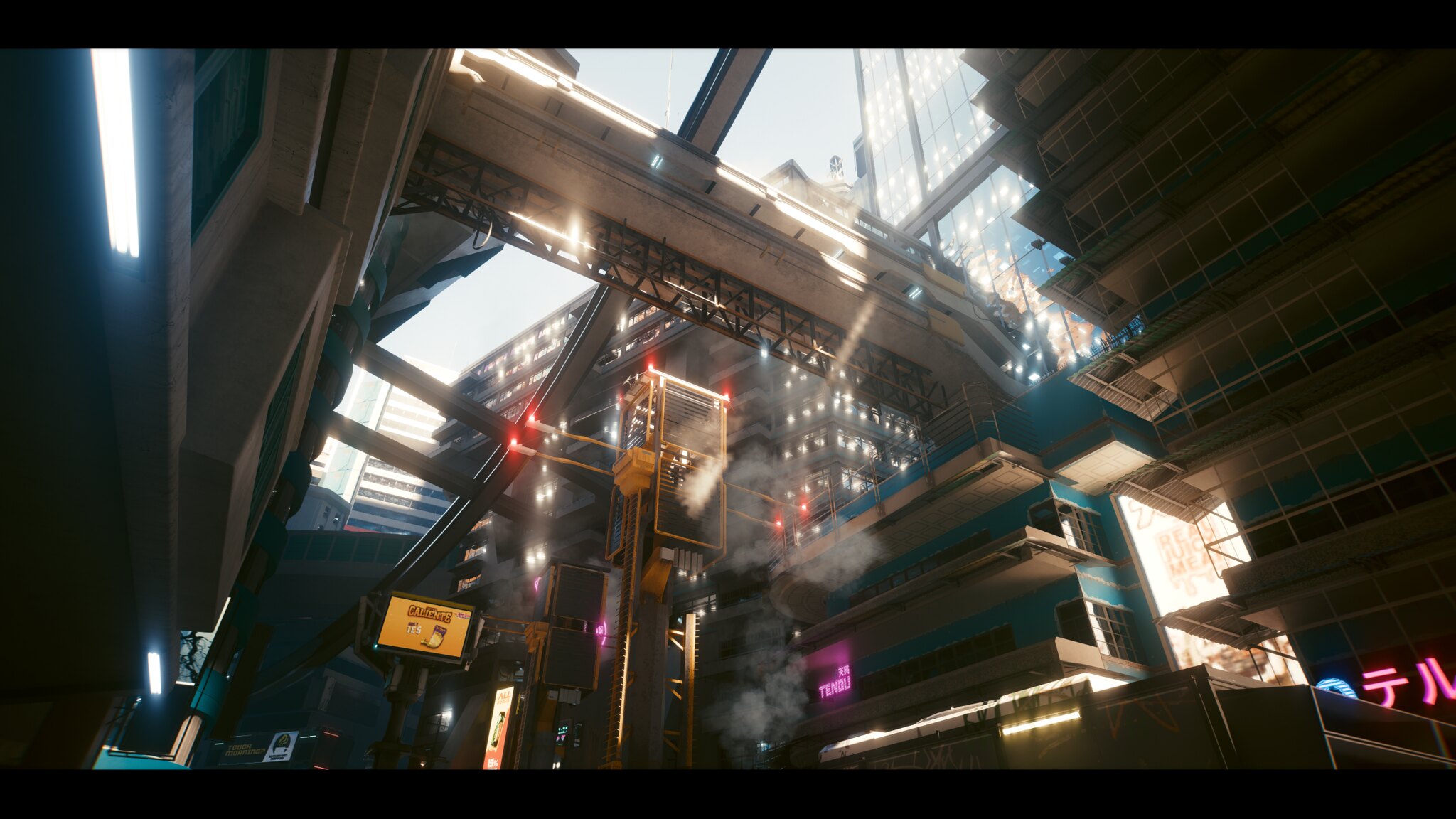The image presents a complex and detailed scene, resembling a first-person perspective screenshot from a video game or a piece of digital artwork. Central to the composition is an exposed, metal elevator encased in a striking yellow cage, featuring a black cage front and positioned on a thin, single metal lift. Flanking the elevator are two mechanical arms with red lights, while a small portion of a yellow ladder runs up its side.

To the right, a segment of a building can be seen, featuring continuous rows of windows paired with numerous small balconies. On the building’s corner, a prominent neon sign in Chinese characters adds a vibrant touch. A distinctive graphic advertisement states "Caliente 1E5" on a yellow banner amid the plethora of illuminated signs, able to catch the viewer's eye from the street below. Fluorescent lights contribute to the cityscape's illumination, alongside various other advertisements and streetlights, although the crosswalk indicators are turned off.

To the left, another building is partially visible, featuring a large rectangular fluorescent light fixture. At the top center of the image, a monorail track slices through the air, conspicuously supporting a seemingly damaged or blown-up bus. The bright, light blue sky overhead suggests a sunny day, casting reflections on the urban scenery below – an array of towering skyscrapers and vibrant neon signs in pink and yellow, defining this bustling cityscape.